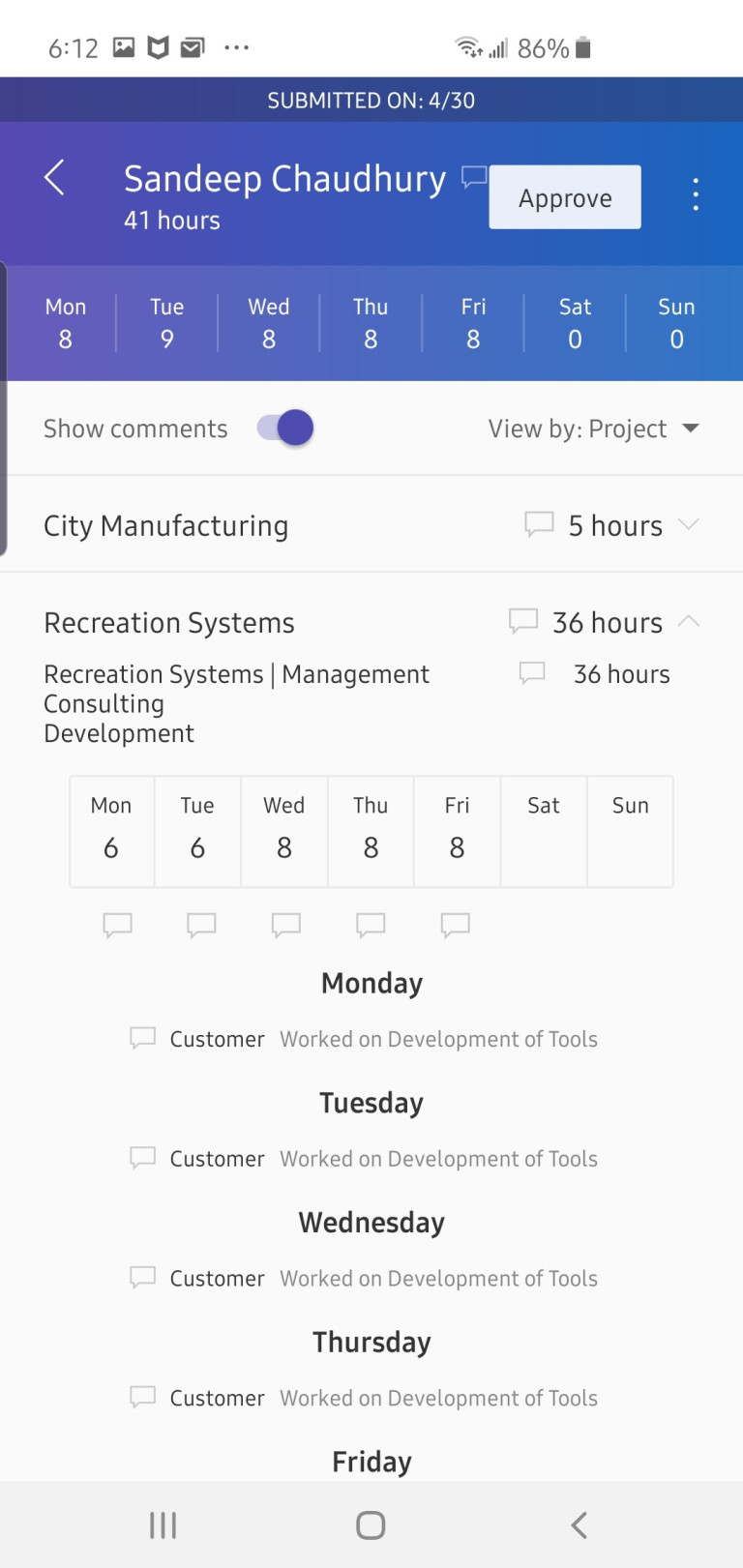The image depicts a detailed job tracking interface for an individual named Sandy Chan, prominently displayed at the top in white text on a blue background. Below Sandy's name, it indicates "41 hours" for the week. To the right side, there is a text box or dialogue caption accompanied by a large white "Approve" button.

The interface breaks down Sandy's weekly hours across different days:
- Monday: 9 hours
- Tuesday: 9 hours
- Wednesday: 8 hours
- Thursday: 8 hours
- Friday: 8 hours
- Saturday: 0 hours
- Sunday: 0 hours

A slider button for "Show Comments" is toggled to the right, indicating that it is active. The current view is "By Projects," which can be changed via a dropdown menu. 

The projects listed include:
- "City Manufacturing" with 5 hours, which can be adjusted.
- "Recreation Systems" under "Management Consultant Development" with 36 hours.

Further details are provided for each project's daily breakdown:
- Monday: 6 hours on customer tool development
- Tuesday: 6 hours on tool development
- Wednesday: 8 hours on tool development
- Thursday: 8 hours on tool development
- Friday: details are cut off in the image

On the left side, there are three navigation icons: three vertical bars, a square, and a left-pointing arrow to go back.

Overall, the interface provides a comprehensive view of Sandy Chan's weekly work schedule, including project hours, daily tasks, and navigation options.